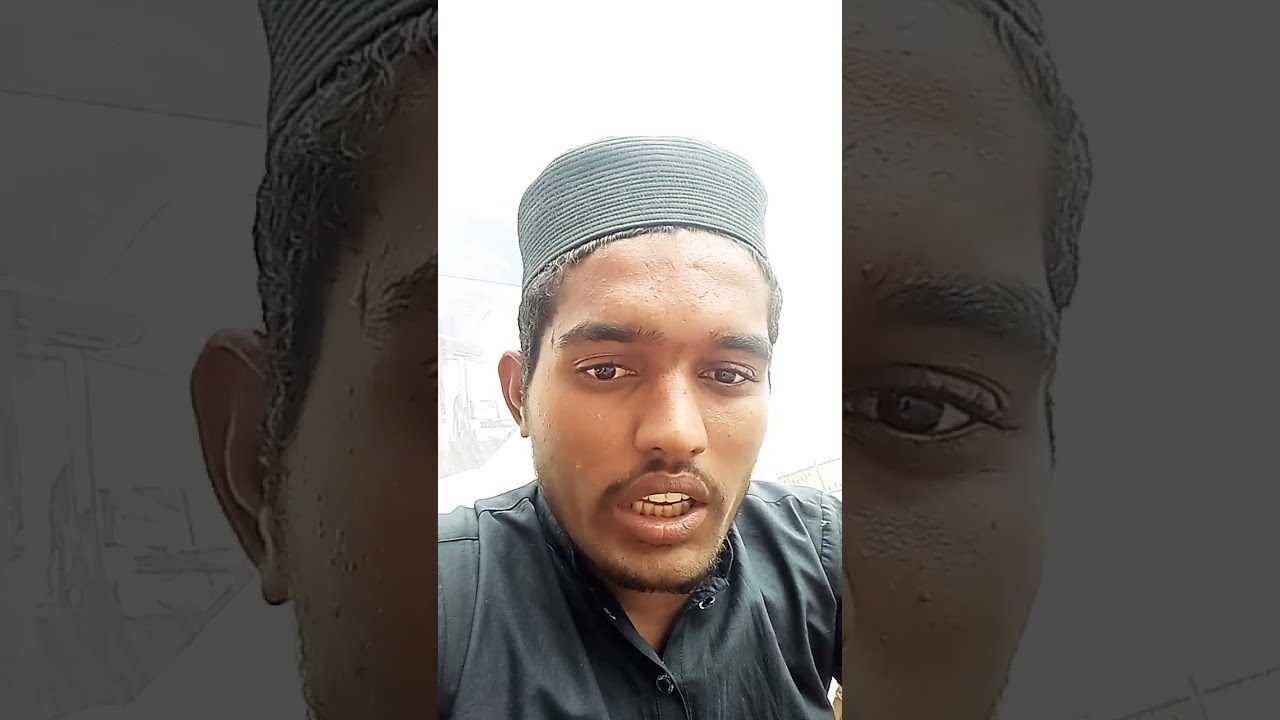The image portrays a close-up of a man of Middle Eastern descent centered in the frame. The background consists of two enlarged and partially shaded sections of the same man's face, showing his ear and part of his face on the left side, and his eye and the other side of his face on the right. The background sections create a stylized, multi-layer effect. The man, with brown skin and straight black hair cut close to his head, is wearing a fez-style, flat-topped hat in black or gray, tilted back to reveal his full forehead. He has thick black eyebrows, brown eyes, a prominent nose, and full lips, parted to show his teeth as if caught mid-sentence. The man sports a thin brown mustache and trimmed chin whiskers. He is dressed in a green button-down shirt with some buttons undone. The colors in the image are predominantly white, gray, black, brown, and green, and there are no other objects or text present. The scene is well-lit, suggesting it was taken outdoors in the middle of the day, perhaps as a selfie intended for social media.